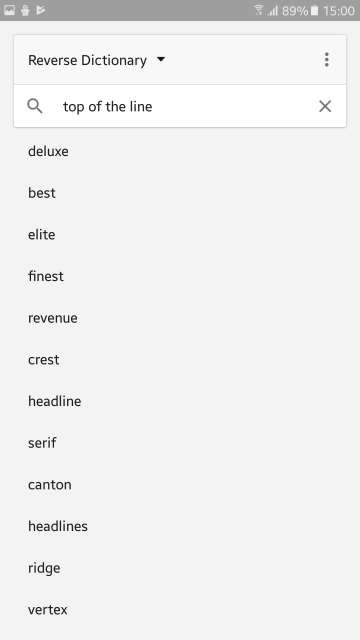The image displays a digital interface. At the top, there's a dark gray border containing indicators for a full Wi-Fi signal, an 89% battery level, and the time displayed as 15:00. Below this border, there's a rectangular box with a light gray top and a white bottom. The top section of this box is labeled "Reverse Dictionary" with a downward-pointing arrow and an ellipsis on the right side. The bottom section features a magnifying glass icon aligned to the left, adjacent to a horizontal line, and an 'X' icon to the right.

Below this interface box, the background is a light gray color. An ordered list of words is displayed vertically from top to bottom: Deluxe, Best, Elite, Finest, Revenue, Crest, Headline, Serif, Canton, Ridge, and Vertex. The right side of the image consists of empty blank space, with no additional elements or descriptions.